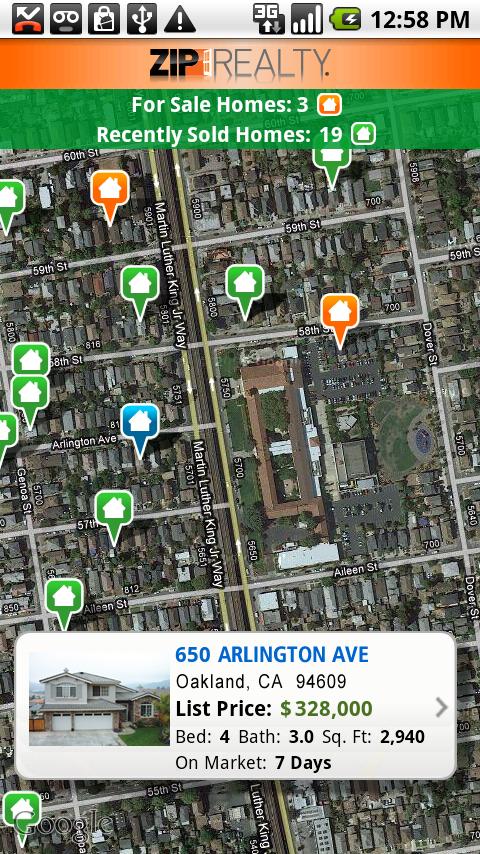A satellite image prominently displays a neighborhood with homes for sale, likely sourced from a real estate website or app. The aerial perspective captures gray and dark rooftops amid patches of visible grass, while streets and home plots are clearly delineated. Various colored pins mark properties on the market: orange, green, and one blue, all adorned with a white home symbol.

The top of the screenshot hints at being captured from a mobile device, showing typical phone icons - voicemail, low battery, 3G signal, signal bars, battery indicator, and the time 12:58 p.m. An orange bar at the display's top reads "Zip Realty," followed by a green bar titled "Home for Sale Homes 3," featuring an orange home pin icon. Another bar below lists "Recently Sold Homes 19" with a matching green pin icon.

The bottom fourth of the graphic includes a white rectangular overlay detailing a specific property: 650 Arlington Avenue, Oakland, California. The list price is set at $328,000 for this four-bedroom, three-bath, 2,940 square foot home that has been on the market for seven days. This information is presented in black and green text beside a small image of the house within the white rectangular overlay.